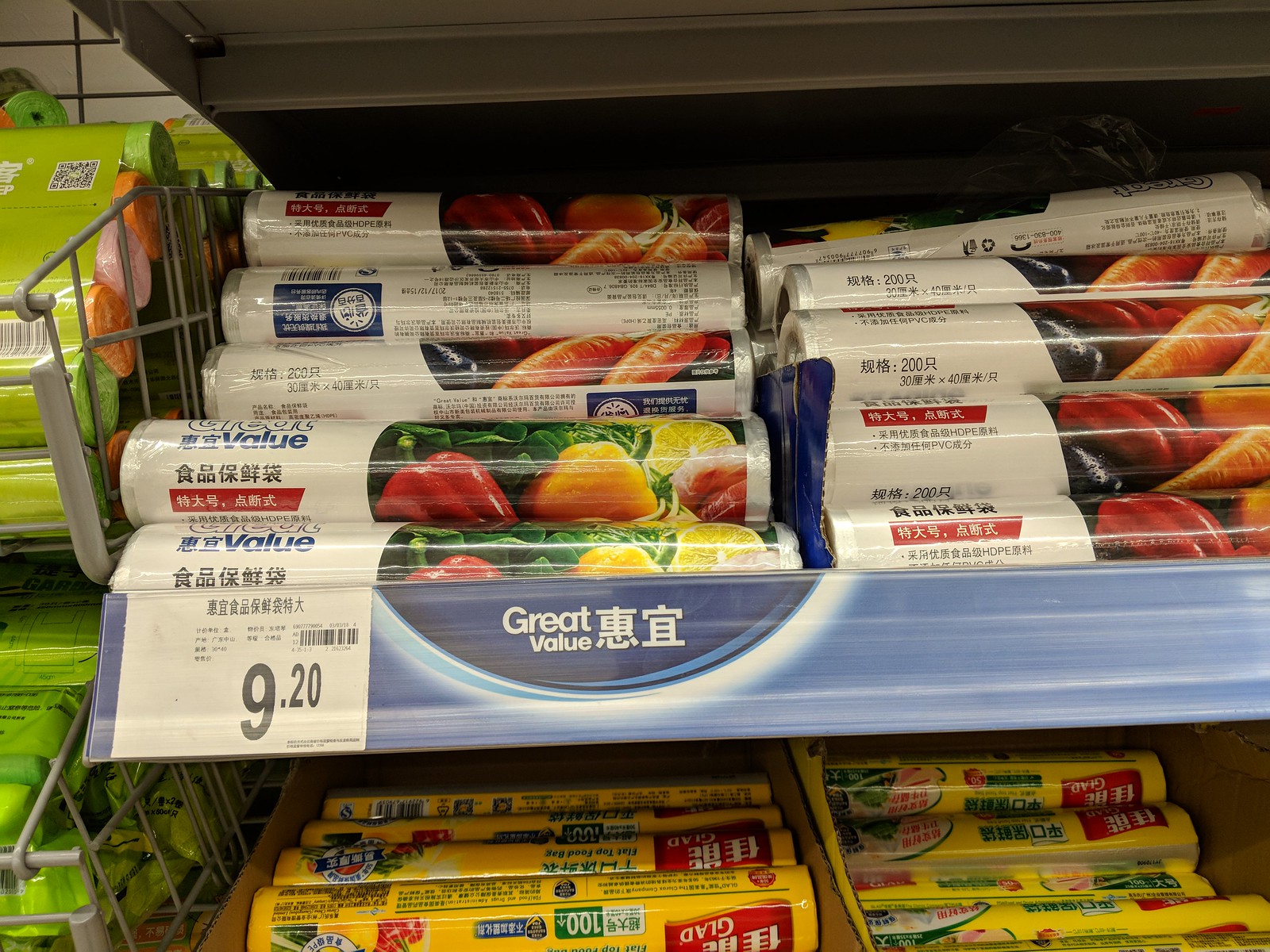In a bustling food store aisle, a section prominently displays Great Value-branded products, likely associated with Walmart. Featured are rolls of Great Value vegetables, their packaging adorned with Asian script, adding an exotic touch. Each roll is wrapped in a clean, white label showcasing vivid depictions of colorful vegetables, including red peppers and possibly yellow peppers. The image captures two well-stocked shelves, prominently showcasing Great Value. To the right, another brand in green packaging is partially visible, highlighting a competitive placement but not drawing focus away from the Great Value products.